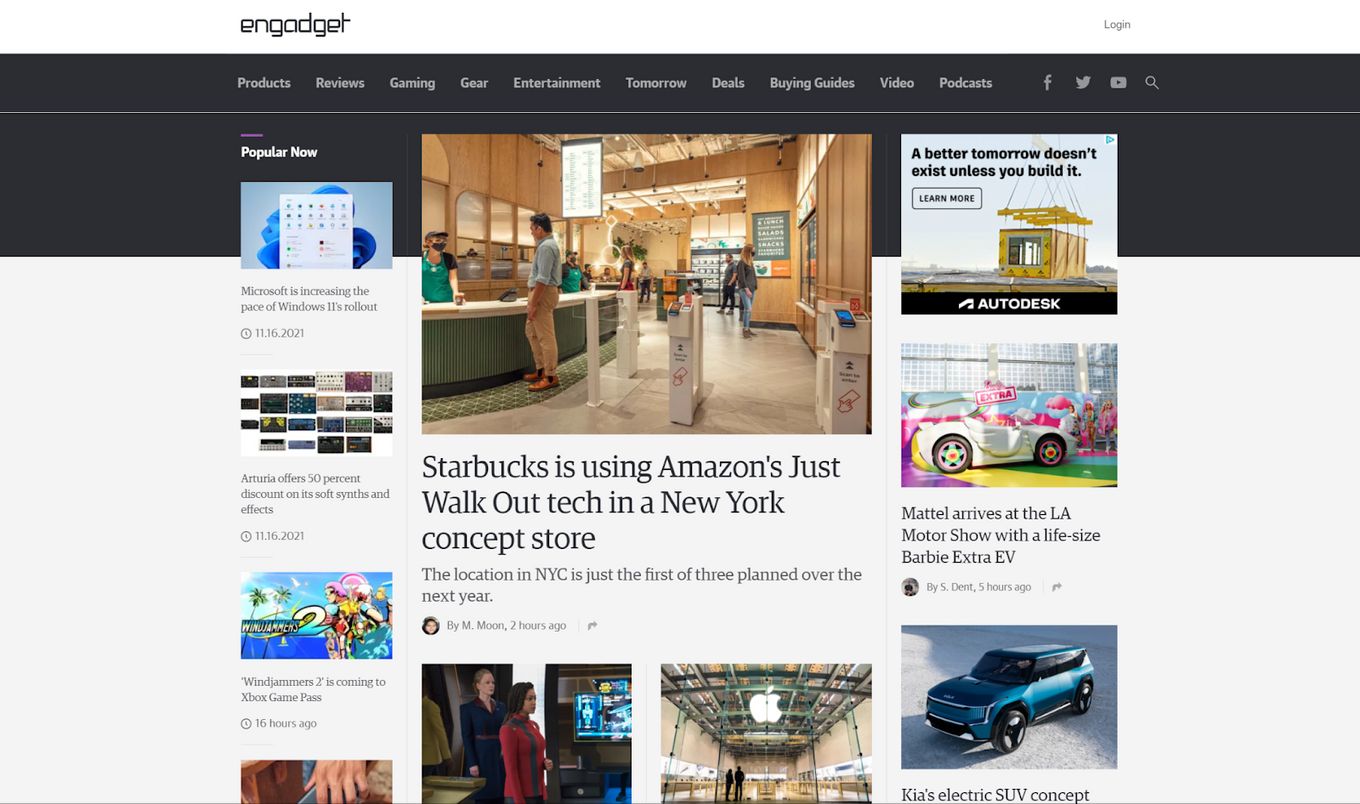The screenshot showcases the homepage of Engadget, a technology-focused news website. In the upper-left corner, the Engadget logo is prominently displayed. A navigation menu runs horizontally below, featuring categories such as Products, Reviews, Gaming, Gear, Entertainment, Tomorrow, Deals, Buying Guides, Video, and Podcasts.

On the left side of the page, there is a "Popular Now" section. It includes a blurry image resembling a computer screen, accompanied by the headline "Microsoft is increasing the pace of Windows 11's rollout," dated 11-16-2021. Below this is another photo with numerous smaller, indistinct images, labeled "Arteria offers 50% discount on its Soft, Synths, and Affects." Further down, there's an image of a video game cover with the text "Windjammers 2 is coming to Xbox Game Pass."

Dominating the center of the page is a large photograph depicting the interior of a business. A counter is visible, staffed by a woman in uniform assisting a man placing an order. Above the counter, a menu is suspended from the ceiling. Additional individuals are seen in the background. Below this central image, a headline reads, "Starbucks is using Amazon's Just Walk Out tech in a New York concept store," noting that this NYC location is the first of three planned openings over the next year.

Further down the page, there are more photos. The first on the left shows two women, while the second features the Apple logo hanging from the ceiling. In the right column, a motivational tagline states, "A better tomorrow doesn't exist unless you build it," followed by the name Autodesk. Below this is an image of a car with the caption, "Mattel arrives at the LA Motor Show with a life-size Barbie extra EV." Another photo of a vehicle follows, captioned "Kia's electric SUV concept."